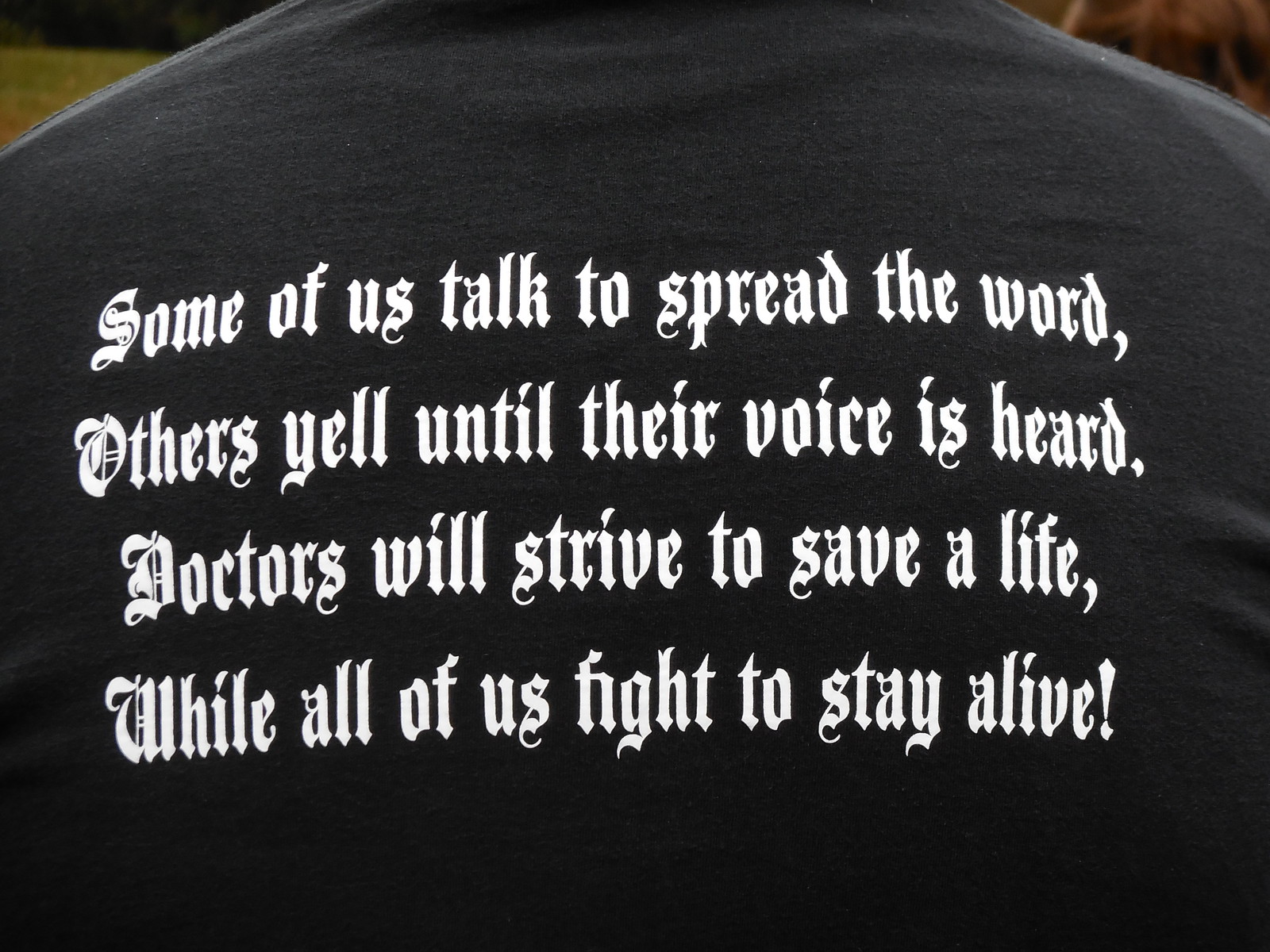The image features a close-up of the back of a dark gray, almost black, shirt adorned with a white, stylized Gothic font. The shirt's poetic text reads:

"Some of us talk to spread the word, 
others yell until their voice is heard. 
Doctors will strive to save a life, 
while all of us fight to stay alive."

This wording is spread across four lines, each beginning with a large, ornate capital letter. The text is roughly centered on the shirt. The shirt's background setting shows hints of a natural landscape, with the top left corner revealing a field with some green grass and possibly trees, while the top right corner displays an amber hue, possibly from the surrounding environment. The photo is taken from the back, solely focusing on the poetic message on the shirt.